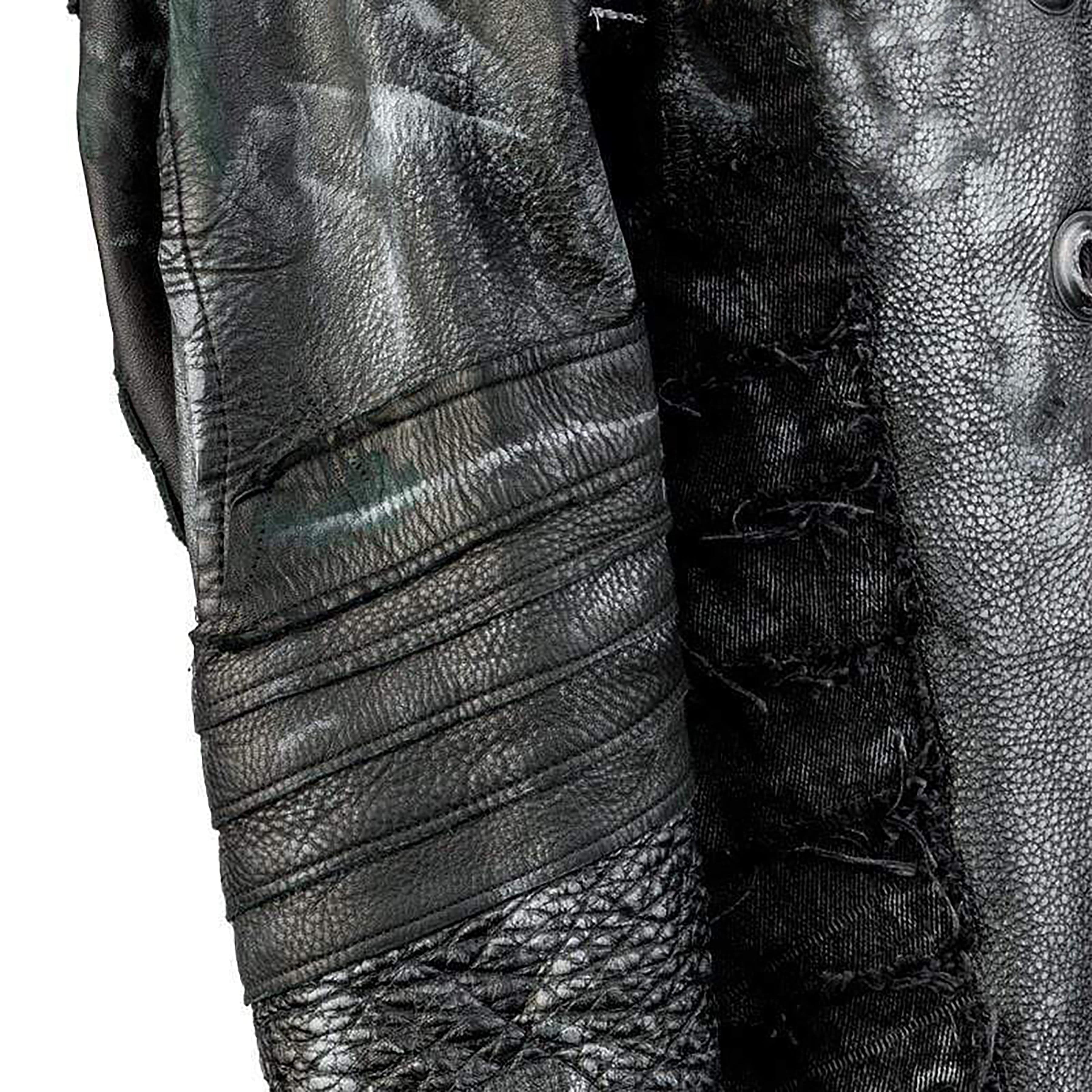The image depicts a black leather jacket that has prominent white age marks, giving it a worn and vintage appearance. The sleeve showcases intricate designs at the bottom and consists of different leather patterns sewn together, offering a textured variety. In the center, there's a slight separation revealing some underlying fabric, possibly jean material, indicating that the bodice might be a combination of leather and denim. A notable detail includes a metal ring used for buttoning, suggesting functional elements within the design. The top left corner of the jacket has a subtle greenish glow. On one section, synthetic strings stretch across in a layered fashion, transitioning into a scaly pattern of small triangles and squares. The right side of the image shows more uniform leather texture with similar small geometric patterns, contrasting with the center's blue jean-like fabric. This detailed close-up captures both the complexity and the aged character of the jacket, blending various textures and designs into a singular garment.